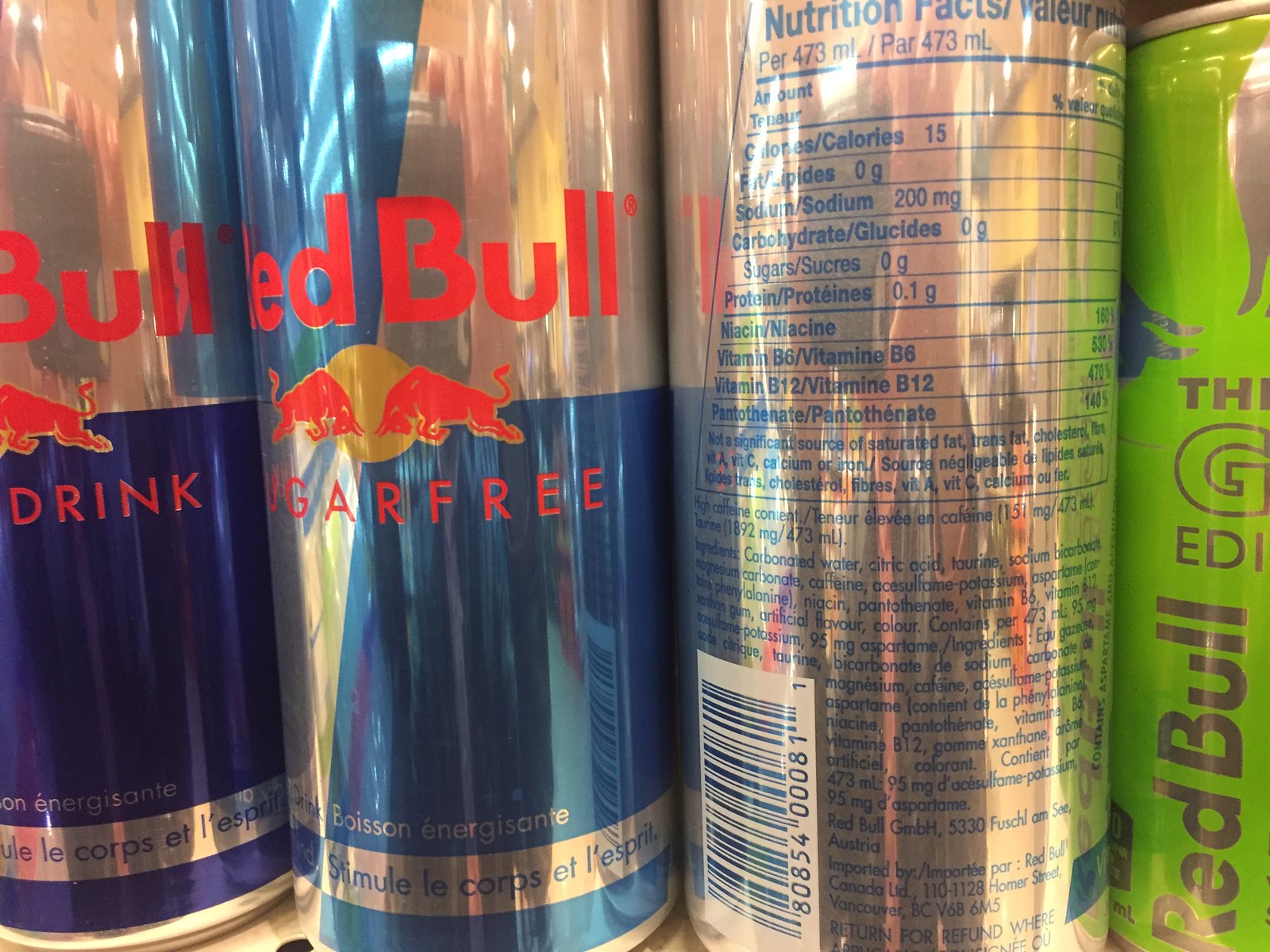This image displays a close-up of four Red Bull cans, each from distinct product lines. Starting from the left, the first can is a standard sugar-free Red Bull, identifiable by its silver and deep royal blue design. The prominent Red Bull logo is set in red letters at the top, with "Sugar Free" written below in matching red font. In the center, two iconic Red Bulls charge towards each other with an orange circle between them. Further details include French text printed in blue on a silver strap line around the can.

The second can, positioned to the immediate right, also shows a similar silver-blue color scheme with the Red Bull logo and "Sugar Free" text. Unlike the others, this can is rotated to display the ingredients and nutritional information, written in blue text on the silver background. This section reveals content such as 15 calories per 473 mL serving and 200 mg of sodium.

The third can, situated further to the right, shares a similar silver facade but emphasizes its nutritional label, which includes a barcode at the bottom. Finally, the fourth can stands out with its lime green color and is slightly shorter. This appears to be a special edition, as indicated by the partial text "EDI" for "Edition" and an embellished "G" symbol. The can's branding features "Red Bull" in silver letters and a subtle bull image at the top.